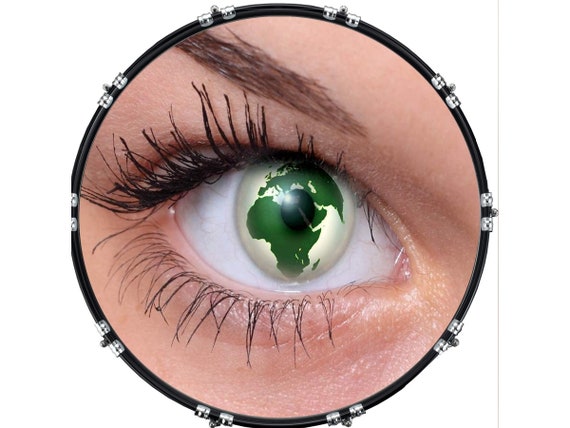In a rounded frame reminiscent of an optometrist's machine, this image captures an extraordinarily detailed close-up of an eye. Surrounded by silver clamps and screw bits, the eye is set against a black circular backdrop. The eye is white with prominent red veins, and its eyelashes are long, dark, and coated with mascara – the top lashes curling upwards and the bottom ones curling downwards. A light brown eyebrow arches above. Fascinatingly, instead of a typical iris, the eye features a green planet resembling Earth, with defined green continents and off-green oceans, and a black pupil at the center. The person's skin around the eye is white, highlighting the sharp contrast and enigmatic beauty of this otherworldly gaze.